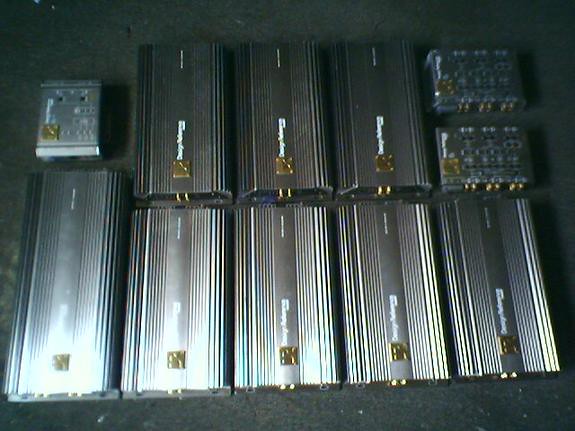The image is a photograph with a black background, focusing on an array of battery packs in various shapes and sizes. In the upper left corner, a small, nearly square, light grayish battery with tiny wires and squares is visible. To its left is a row of three identical black rectangular batteries, each featuring gold squares and prongs at their ends. At the far right, two grayish square batteries, stacked one on top of the other, display three sets of gold prongs at their bases. Among these, on a gray-colored surface, lies the largest battery—a long rectangular black one with a gold square and prongs at its bottom. Below this, four identical black batteries with gold squares and prongs are arranged in a row. The overall assemblage, potentially comprising some sort of converters or amplifiers, lacks a clear sense of scale due to the ambiguous context. The dim lighting, possibly reflecting the camera's flash, adds to the metallic sheen and partially obscures the finer details, including white writing on the faces and tops of the items, making it challenging to definitively determine their precise function.